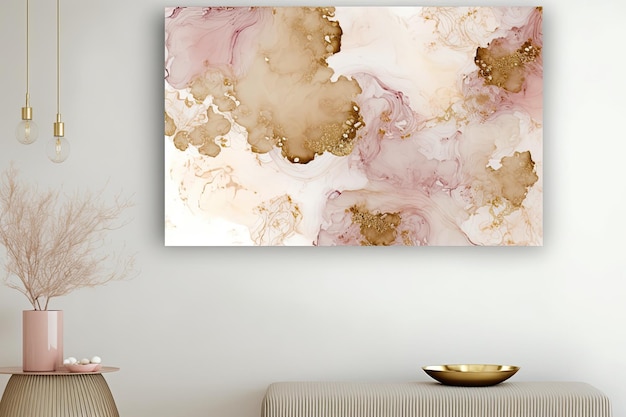The image captures a modern and stylish room with a neutral color palette accented by millennial pink, gold, and bronze tones. Dominating the scene is an abstract canvas on a gray wall, featuring splotches of tan, brown, pink, dark pink, and cream, resembling marbled watercolor or ink blots. Below the painting, a black and white striped ottoman supports a golden dish. To the left, two clear bulb hanging light fixtures illuminate a small pink planter containing feathery, nude-colored, fluffy plants, all situated on a ledge or side table. The overall composition of the room exudes a contemporary and sophisticated aesthetic, captured in what appears to be a professional photograph of a stylishly decorated interior.